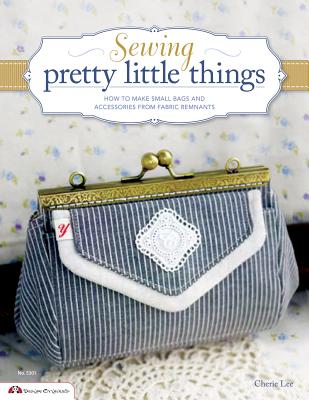This image appears to be the cover of a magazine or instructional book focused on sewing. The title, prominently featured within a blue-bordered white text box at the top center, reads "Sewing" in cursive, followed by "Pretty Little Things" in blue text, and then "How to Make Small Bags and Accessories from Fabric Remnants" in smaller blue text. The background is adorned with a delicate white fabric printed with tiny blue cornflowers. Dominating the bottom half of the cover is an eye-catching blue and white striped corduroy coin purse, featuring a decorative white diamond design on the front. The purse boasts a gold clasp at the top and appears to be resting on a white lace doily, adding to the overall charming and crafty aesthetic of the cover. The author of this instructional guide is Sherry Lee.